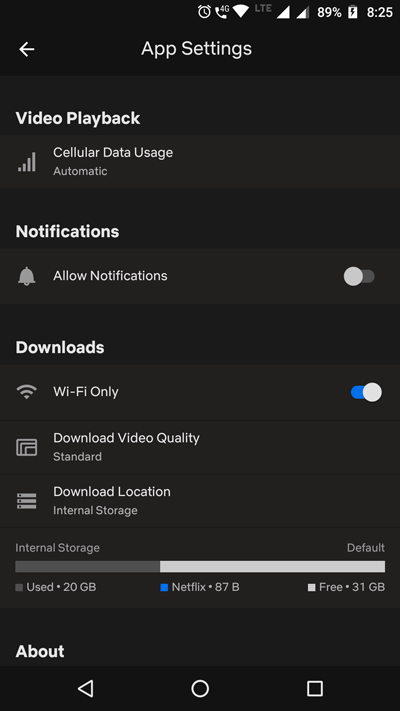A detailed screenshot from a mobile phone interface with a dark theme. The top section includes standard mobile status icons: a Wi-Fi signal, two different SIM card indicators, an 89% battery level, and the current time displayed as 8:25. Below this, centralized app icons include a back arrow for navigation.

Primary content shows various settings segmented into distinct rows of slightly differing shades of black and dark gray. The first setting pertains to **video playback** with a cellular data usage indicator and cellular icon. Following that are **notifications** settings, marked by a bell icon and an "Allow notifications" toggle set to off. The **downloads** section features a Wi-Fi icon with a "Wi-Fi only" download setting turned on (indicated by a blue slider). It also notes "Download video quality: Standard" alongside a small square icon, and "Download location: Internal Storage."

At the bottom is a dual-colored bar with dark gray on the left and near-white on the right, providing storage details: "Internal storage used: 20 GB," "Netflix: 87 bytes," and "Free: 31 GB," with "Default" labeled above it—likely the default storage location. 

The left section includes an "About" option, and below that are the navigation options: a back button, a round home button, and a square recent apps button. The absence of a scroll bar, owing to the black background, suggests the possibility of more settings below the visible portion.